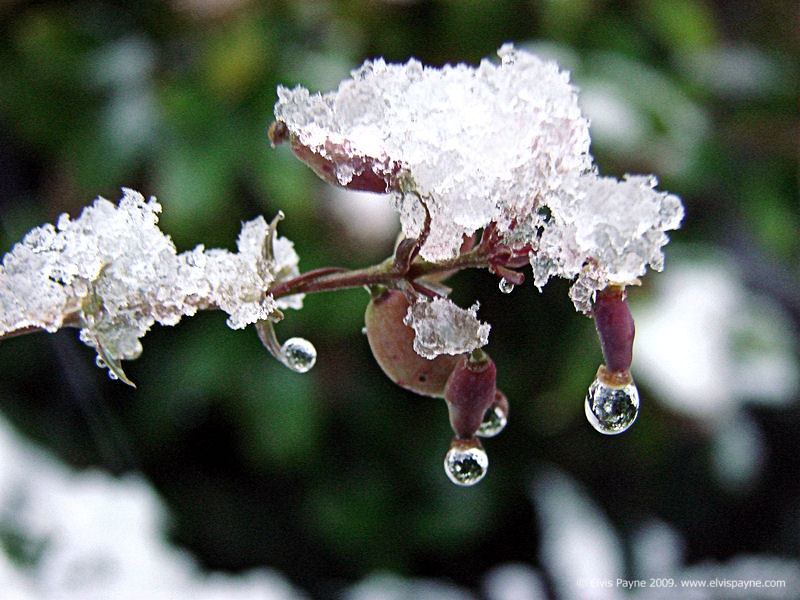In this photo, a magenta-colored plant branch is prominently featured, extending diagonally from the upper left to the center of the image. The vivid branch, interspersed with magenta buds, stands out against a wintry backdrop. The buds, positioned two on the top and two on the bottom of the branch, are adorned with beads of water that have frozen into clear, crystalline droplets. These spherical droplets are heavy and appear on the verge of bursting. The ice encapsulates the branch almost completely up to the dry section near the center. Three of the flower buds on the underside of the branch display these large, frozen bubbles, contributing to the serene yet fragile beauty of the scene. The overall effect is a vivid display of winter’s icy grip on the otherwise colorful and lively branch.